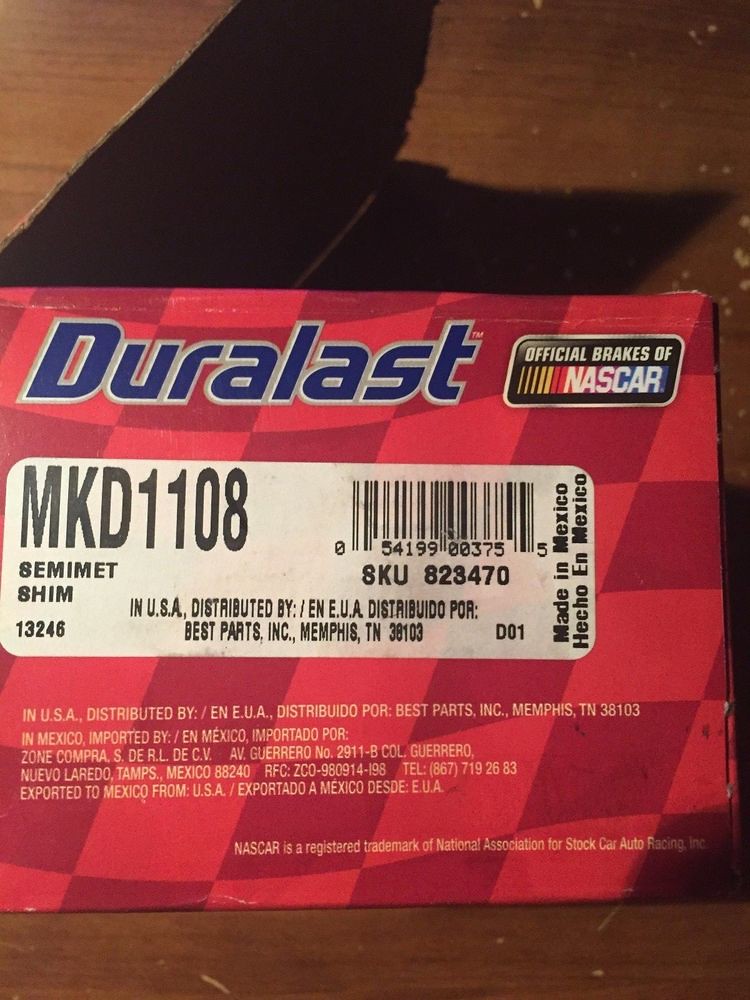This detailed color photograph showcases a product package for DuraLast, the official brakes of NASCAR, set against a background of a brown wooden table. The package features a vivid red and black checkered design. The text "DuraLast" is prominently displayed across the top in blue letters with white edges. Below this, a black rectangle contains the text "official brakes of NASCAR" in white font, accompanied by the NASCAR logo which incorporates blue, purple, red, and yellow colors. A prominent white shipping label in the center of the package reads "MKD1108SEMIEMETSHIM," and additional smaller alphanumeric codes such as SKU 5419900375 and 823470 are included, along with a Scantron barcode. The packaging also features white text stating "NASCAR is a registered trademark of the National Association for Stock Car Auto Racing," as well as details indicating that it is made in Mexico and distributed or exported to Mexico from the USA.